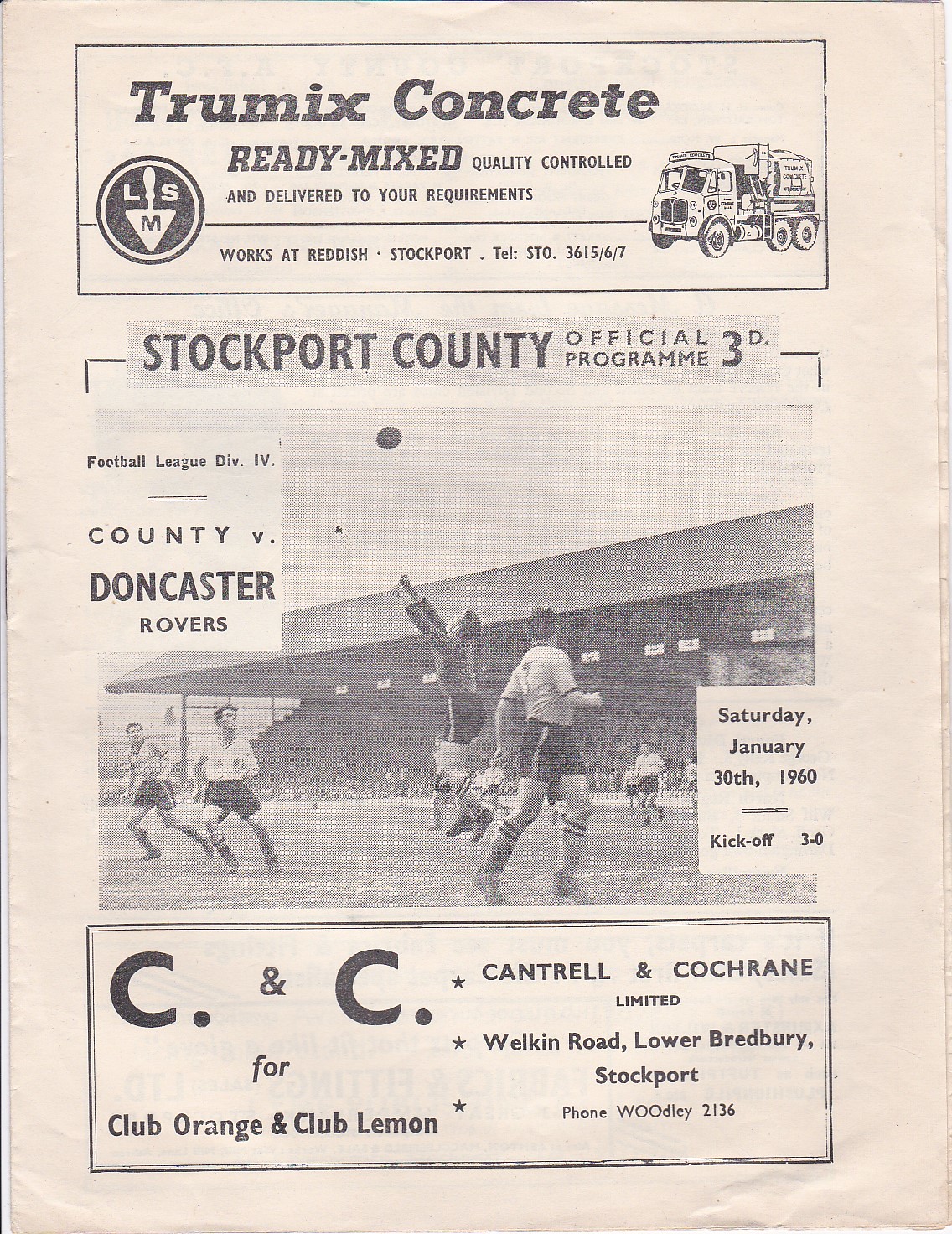This vintage page from the Stockport County Official Program, priced at 3d, showcases a dynamic blend of sports and advertisements from 1960. Dominating the top section is an ad for "TrueMix Concrete," emphasizing their ready-mix, quality-controlled services, based in Reddish, Stockport, contactable via telephone at STO 3615/6-7. The ad features a logo with a trowel marked "LSM" on the left, and an illustrated cement mixer truck on the right.

Beneath this ad lies a nostalgic black-and-white photograph capturing an intense moment in a soccer match with players contesting the ball. The caption boldly announces: "Football League Division 4: County vs. Doncaster Rovers." Mark your calendars for this event on Saturday, January 30, 1960, with a kickoff at 3:00 PM.

At the bottom, a second advertisement promotes Cantrell and Cochrane Limited's beverages, "Club Orange" and "Club Lemon," located on Welkin Road, Lower Bradbury, Stockport. The contact number for this refreshing sponsor is Woodley 2136.